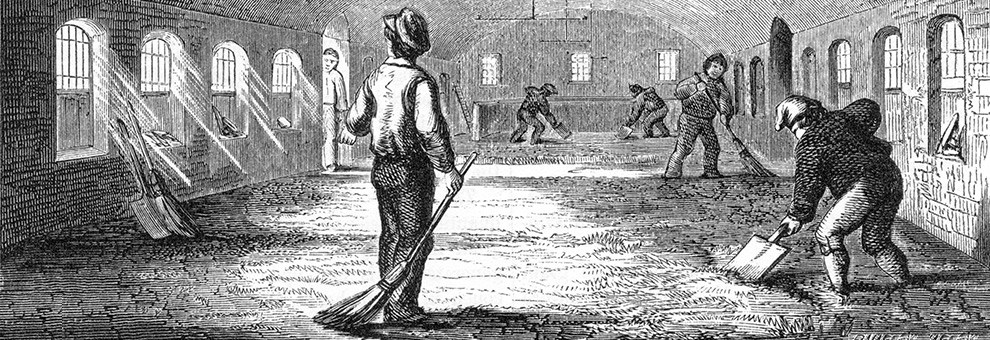The image is a detailed black-and-white illustration of a large, old-fashioned facility, likely a brewery from an 1853 poster. It features a wide-angle, horizontal view of an expansive, brick-walled interior filled with several men at work, all dressed in period attire from the late 18th to early 19th century. Along the left wall, there are four arched windows allowing sunlight to stream through, illuminating the scene. The four arched windows have black iron gates, with shovels and other cleaning tools leaning against this wall. The central figure, located slightly left of center, stands with his back to the viewer. This man is dressed in a cap, white shirt, and dark trousers, and holds a broom in his right hand while gazing towards the windows. 

In the background, there are additional men engaged in various tasks; two men can be seen shoveling and raking the floor, their postures suggesting laborious activity. To the right, another older man in a dark shirt and lighter britches, wearing a distinctive French peaked cap, is bent over a shovel, mucking the area in front of the stalls. Behind him, other figures continue the work, raking hay and cleaning. The far wall in the deepest background has three more arched windows, and a stack of hay is visible. This detailed illustration captures the bustling, industrious atmosphere of the facility, rendered in a vintage, black-and-white lithograph style.